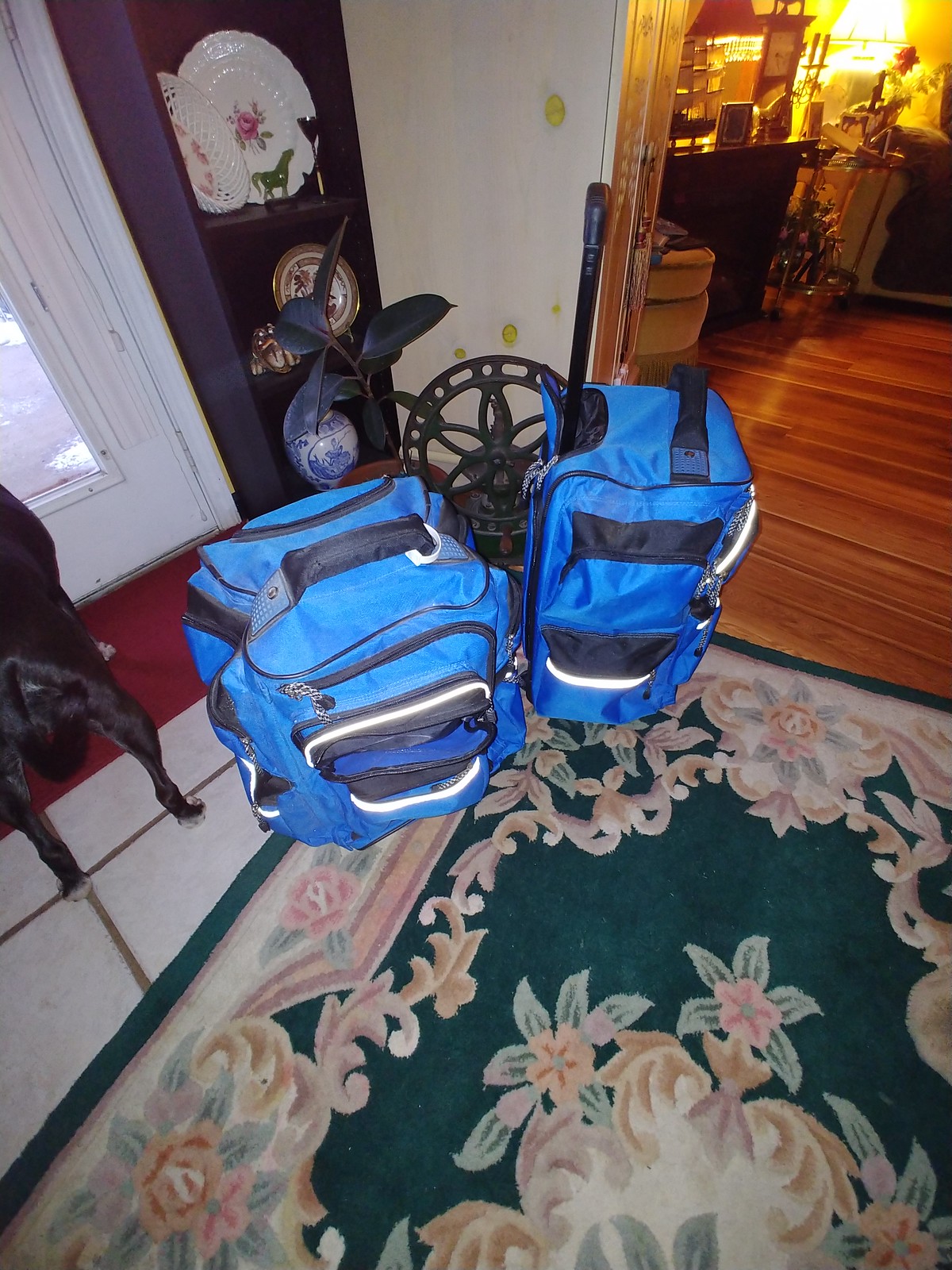This image showcases a vibrant and eclectic room, with various colors and textures. At the center, two pieces of blue luggage—comprised of a backpack and a rolling suitcase with multiple pockets—are placed side by side, ready for travel. The luggage bags feature black zippers and handles, with the suitcase's handle in an upright position. They rest on an ornate green area rug decorated with floral patterns in pink, white, and light green tones. A partially visible black dog stands beside the luggage, gazing towards the door or window.

To the left, there's a red welcome mat lying on a white tile floor, adjacent to a light gray wall. The room boasts a mix of décor elements, including a prominent purple cabinet displaying white ceramic dishes with floral prints, and a blue-and-white mosaic vase. A black bookshelf filled with plates enhances the eclectic ambiance of the space.

In the background, another room can be seen through an open doorway. This room features a brown wooden floor and a dark brown cabinet adorned with flowers. The overall setting appears slightly cluttered yet inviting, with various decorative items and a light in the corner casting a warm glow over the scene.